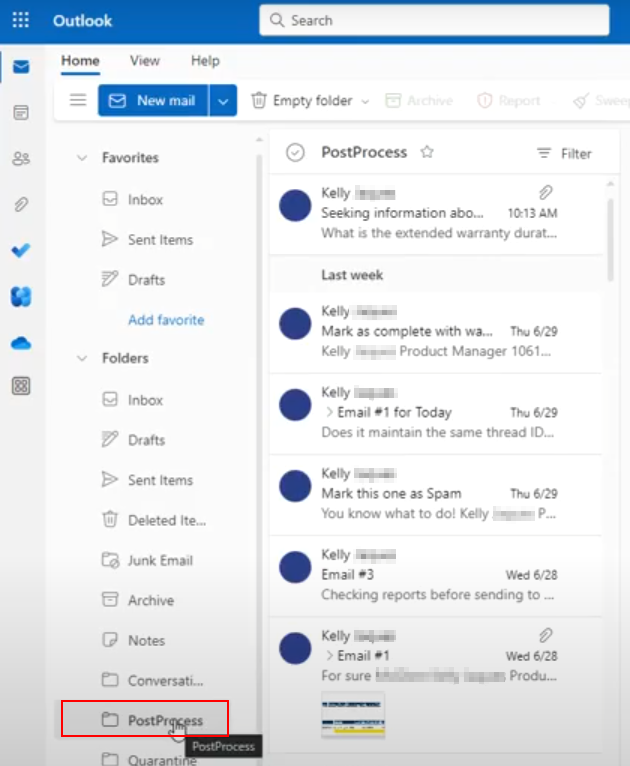A screenshot of an Outlook email web page is presented. At the top of the page, a search bar is prominently displayed. Along the left sidebar, several icons are visible from top to bottom, representing different functionalities: an envelope for email, a person silhouette for users, a pushpin for pinned items, a checkmark, a cloud, and two indistinct icons resembling a cluster of five blue balls and a black square with four colored circles. 

The main navigation tabs across the top include "Home," "View," and "Help." Directly beneath these tabs are options for creating new mail, accessing a drop-down menu, an empty folder icon, a trash can icon, and a "Favorites" section.

The email folders listed are: Inbox, Sent Items, Drafts, Add Favorite, Folders, Inbox, Drafts, Sent Items, Deleted Items, Junk Email, Archive, Notes, Conversation, and Post Process. A specific folder is highlighted in red, labeled "Quarantine."

In the main email section, several emails are listed, all from a sender named Kelly. The emails cover topics such as extended warranty duration, with prompts to mark as complete or spam. The timeline indicates emails received last week and today, with varying subjects and actions suggested for each email from Kelly.